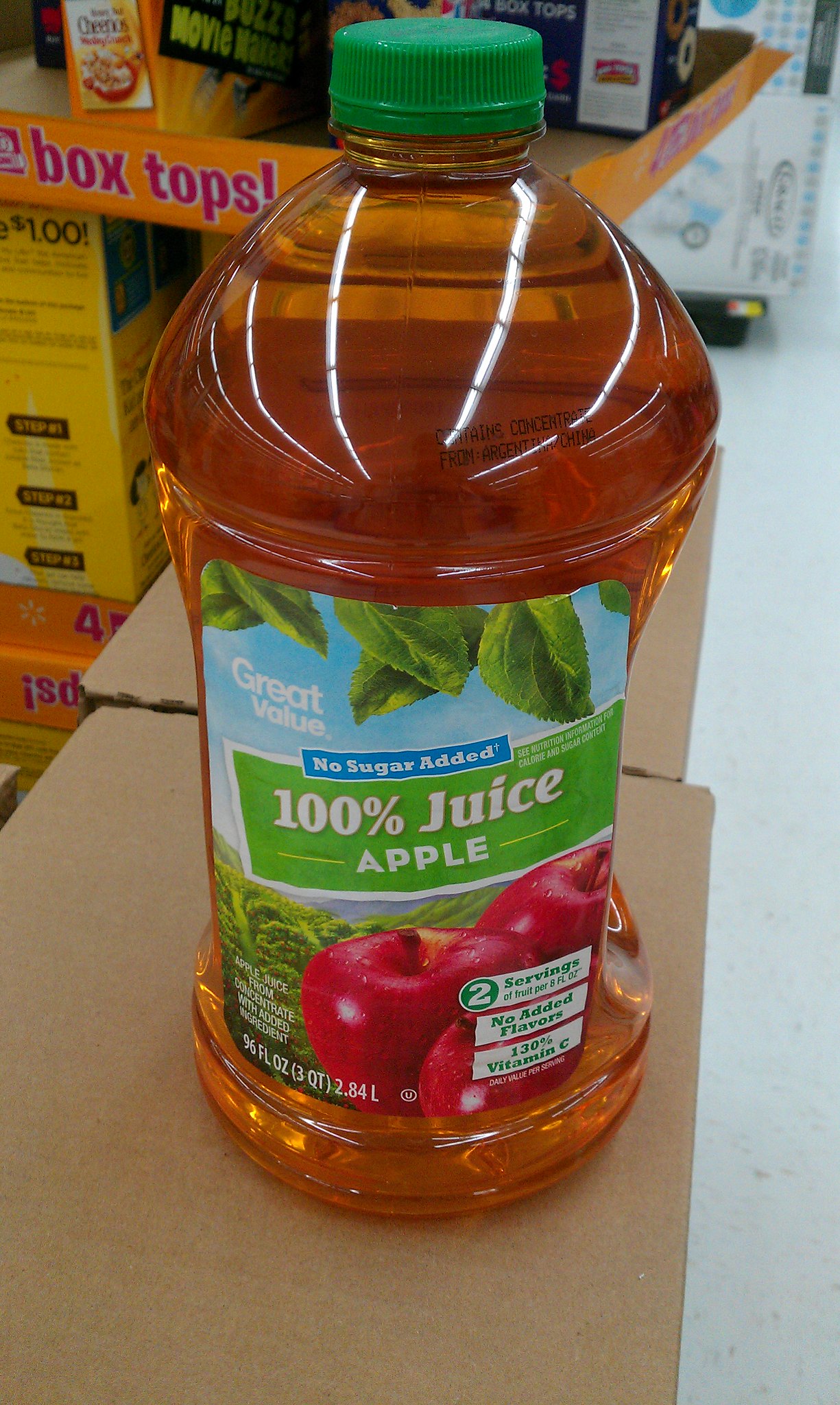This image captures a 96 fluid ounce Great Value brand apple juice bottle, prominently displayed on a box within what appears to be a Walmart store. The bottle is full to the top and sealed with a green cap. Its label is vividly detailed, featuring a picturesque blue sky backdrop with green trees and leaves at the top, and three dewy, red apples at the bottom, emphasizing the freshness and appeal of the juice. Text on the label highlights that it is 'No Sugar Added, 100% Apple Juice,' providing two servings of fruit per eight fluid ounces, containing no added flavors, and offering 130% of the daily recommended Vitamin C intake. The bottle has a user-friendly design with concave sides for easy gripping. The scene is set against a background of store displays, including boxes of cereal and other food items, giving the impression of a typical Walmart sales floor or potentially a donation drive setup due to the arrangement of the other boxes in the image.